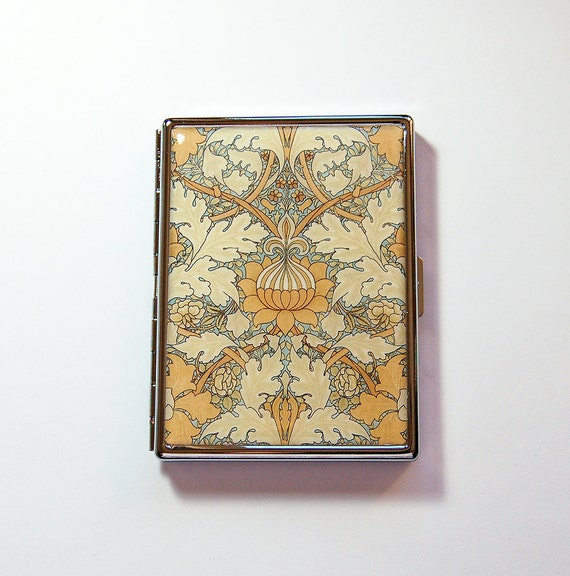The image depicts a vintage cigarette case—or possibly a business card holder—set against a solid white background. The case is crafted from a gold-toned metal, featuring a detailed, enameled Art Deco design on its front. The intricate artwork includes a central round orange blossom, with stylized petals and vines in light orange, tan, and cream hues, branching out elegantly. Adding to its sophistication, the design incorporates delicate black pinstriping and other floral elements, set on a beige background.

Notably, the front image also showcases the stylized faces of two ladies, adorned with elaborate headdresses that resemble plumes of feathers, evoking a sense of theatrical glamour. The surrounding feathers and potential show outfits further emphasize the Art Deco influence.

The case is bordered by metal, with a distinctive gold clasp on the right-hand side for opening, and a line of small hinges on the left, indicating its functionality. The meticulous craftsmanship and ornate design make it a striking and well-preserved piece.